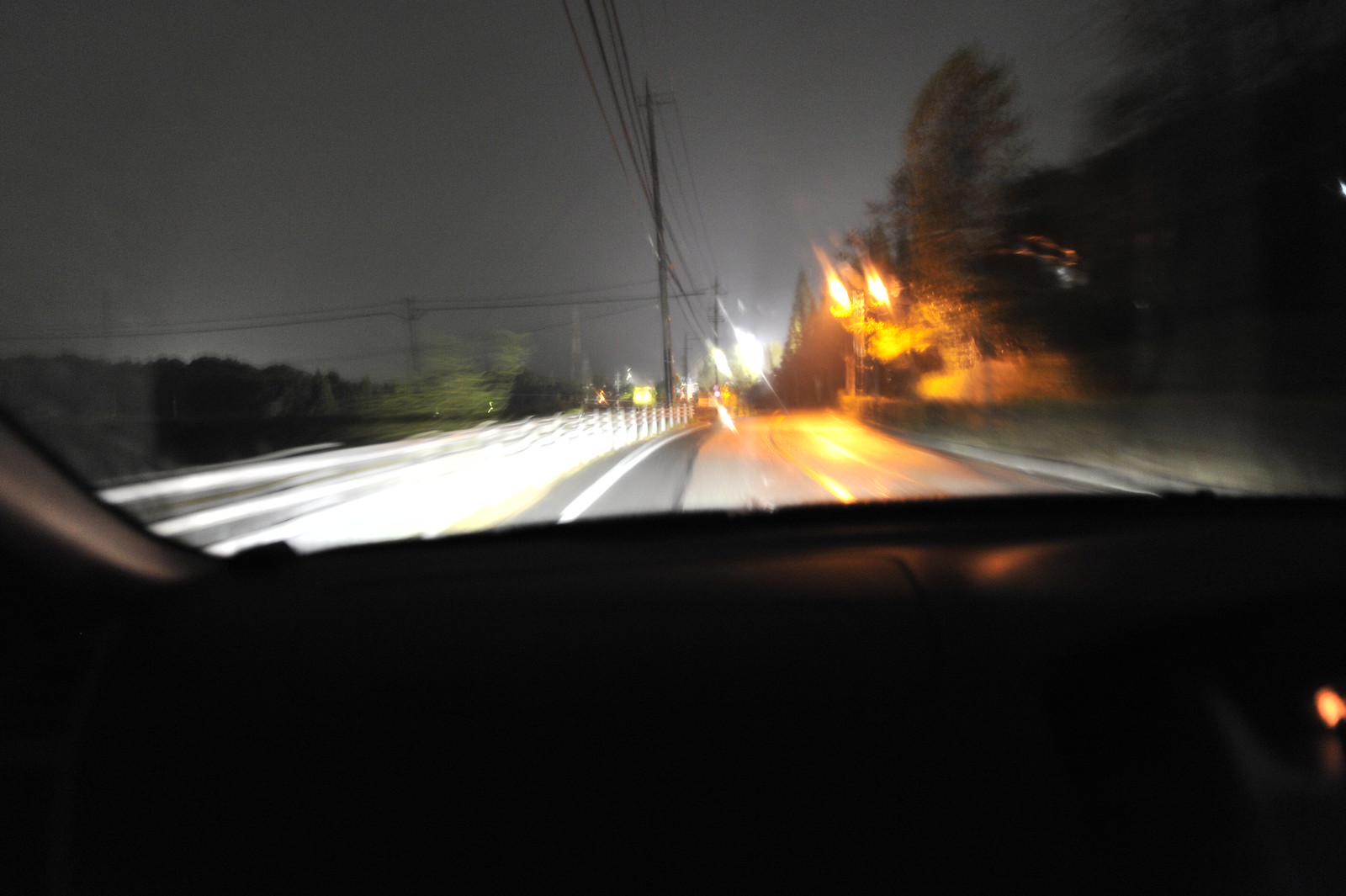This blurry, wide-angle photograph captures a nighttime scene viewed through a vehicle's windshield, though it's unclear if it's the front or rear window. The night sky is an impenetrable darkness, punctuated by a bright light source to the right, casting reflections on the wet street below. The background is a haze of indistinct shapes, suggesting movement and activity. Telephone poles with wires stretch across the center, while blurred headlights from oncoming traffic pierce the gloom. To the far right, the silhouettes of trees are barely discernible. The image, dark and indistinct, conveys a sense of motion and the obscured clarity that comes with nighttime travel.